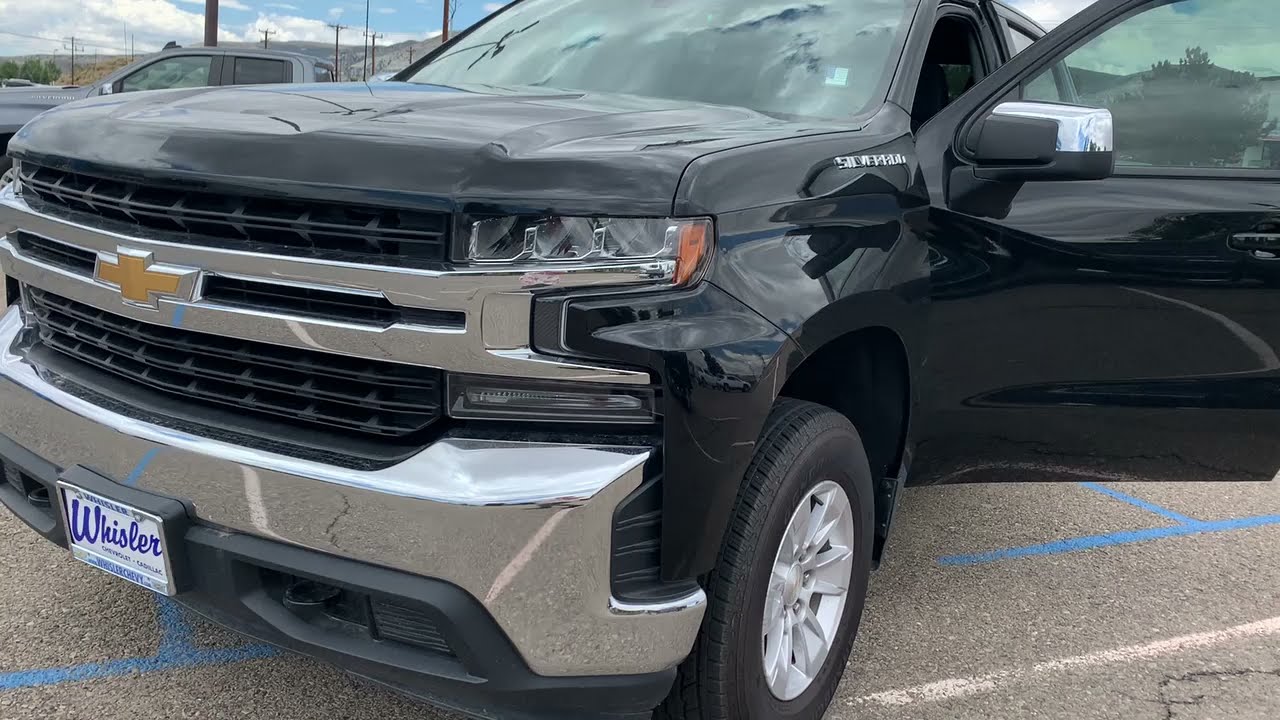This medium shot photo captures a shiny black Chevrolet pickup truck from the front left corner, set outdoors in what appears to be a dealership parking lot. A prominent feature of the truck is the gold Chevy logo on the silver front bumper, paired with the name "Silverado" likely in silver lettering. The truck bears a white license plate with blue text reading "Whistler," indicating it may currently be unregistered and possibly part of the dealer's inventory. The driver's side front door is open, and while it appears there might be a dent, it could just be reflections creating this illusion. The vehicle is positioned on gray pavement marked with blue and white parking lines, and visible behind it is the roof of another gray vehicle. In the distance, the background includes items like poles, phone posts, and hints of natural landscapes such as mountains, suggesting a possible West Coast location like Nevada or California. Above, the sky features a mix of blue and gray clouds, enhancing the outdoor dealership setting.